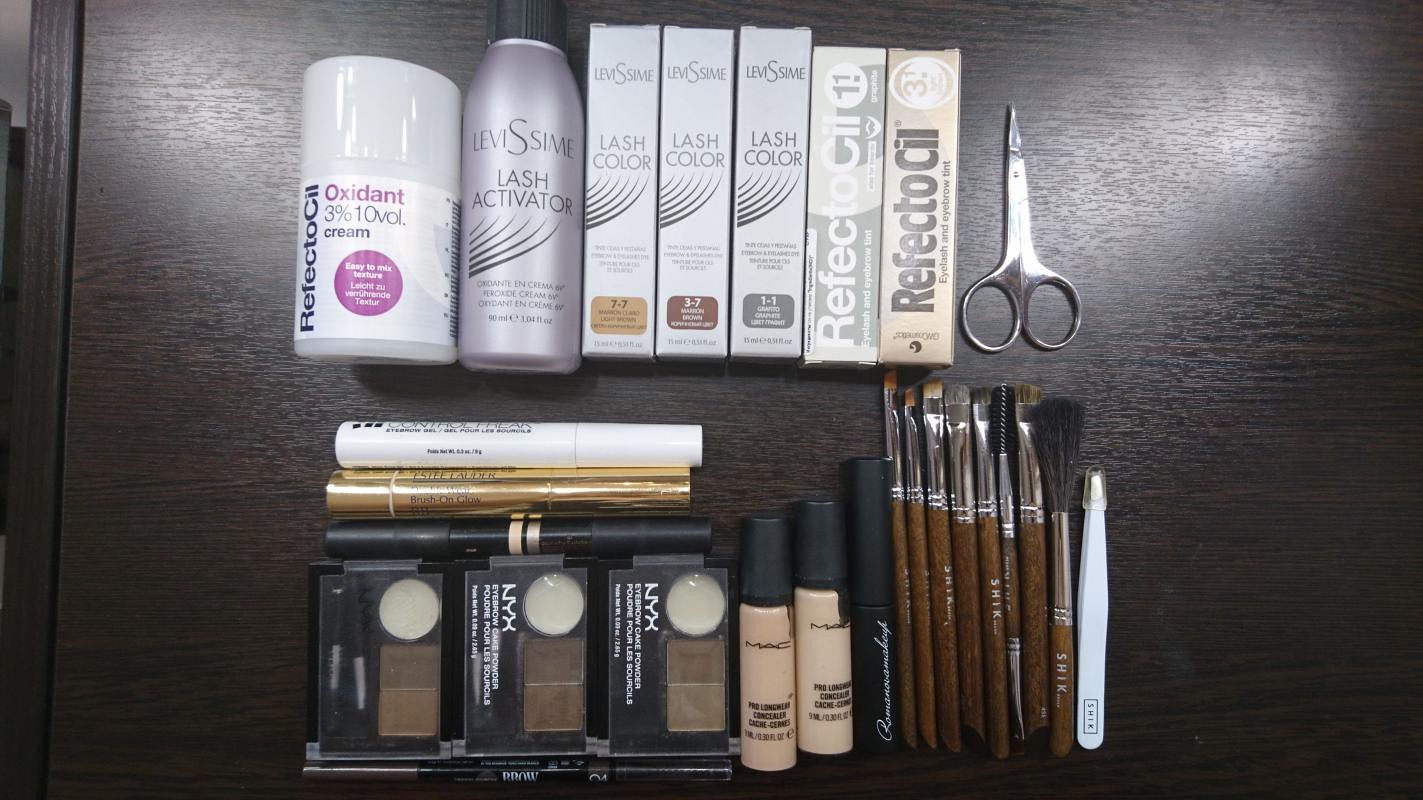Indoor color photograph taken from a top-down perspective of a brown tabletop, showcasing an arranged collection of beauty care products. 

**Top Row:**
- The first two items, positioned left of center, are cylindrical containers. The left one is labeled "Oxidant" in purple lettering, and the right one is marked "Lash Activator" in silver text.
- Following these are five vertical rectangular boxes. The first three are gray and display "Lash Color" in capital letters.
- To the right of the gray boxes is a product with the label "Refectocil" in vertical lettering.
- At the far right of this row, there is a small pair of silver trimmers with a very small cutting edge.

**Bottom Row:**
- This row begins with a collection of mascara tubes placed on top of three black rectangular makeup kits.
- To the right are two round bottles, presumably containing foundation, though the labels are difficult to decipher.
- Finally, at the far right is a collection of seven or eight makeup brushes with brown handles and silver tips. The brush bristles range in color from light brown to dark brown. Next to the brushes is a pair of white tweezers.

The image is well-focused, allowing detailed observation of the items, which appear to be typical beauty products used for facial makeup.